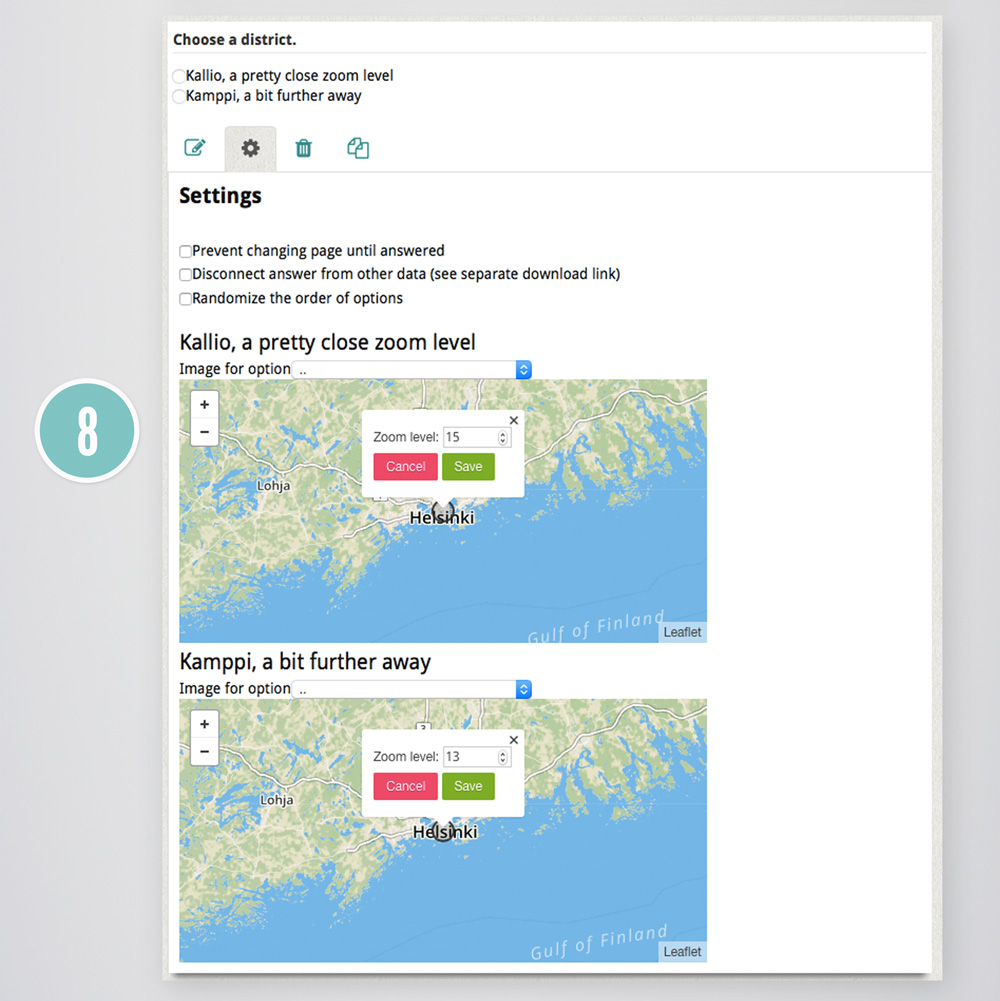The image features a gray background with a layout detailing several UI elements. On the left, there is an icon consisting of a white circle filled with a mint-green to teal gradient, inside of which is a bold, white number "8". 

The main content area, a form or a page, is headed by the text "Choose a District" in a small, black font. Directly below this are two options in smaller black font: "Calio," described as having a very close zoom level, and "Campy," described as having a slightly further zoom level. 

Below these descriptions, a set of four icons is aligned horizontally, each representing different functions: a drawing tool, settings (currently selected), a trash can, and an option for managing multiple pages.

The settings section, marked by the bold word "Settings," includes three checkbox options: "Prevent changing page until answered," "Disconnect answer from other data (see separate download link)," and "Randomize the order of options."

Under the "Calio" option, a close zoom level displays an image showing Helsinki and the surrounding coastline along the Gulf of Finland. The zoom level here is adjustable, currently set at 15, with clickable options to increase or decrease the level. There are also "Cancel" and "Save" buttons.

The "Campy" option, described as a bit further away zoom level, includes an image placeholder and adjustable zoom level, set at 13. Similar to "Calio," there are "Cancel" and "Save" buttons available for user interaction.